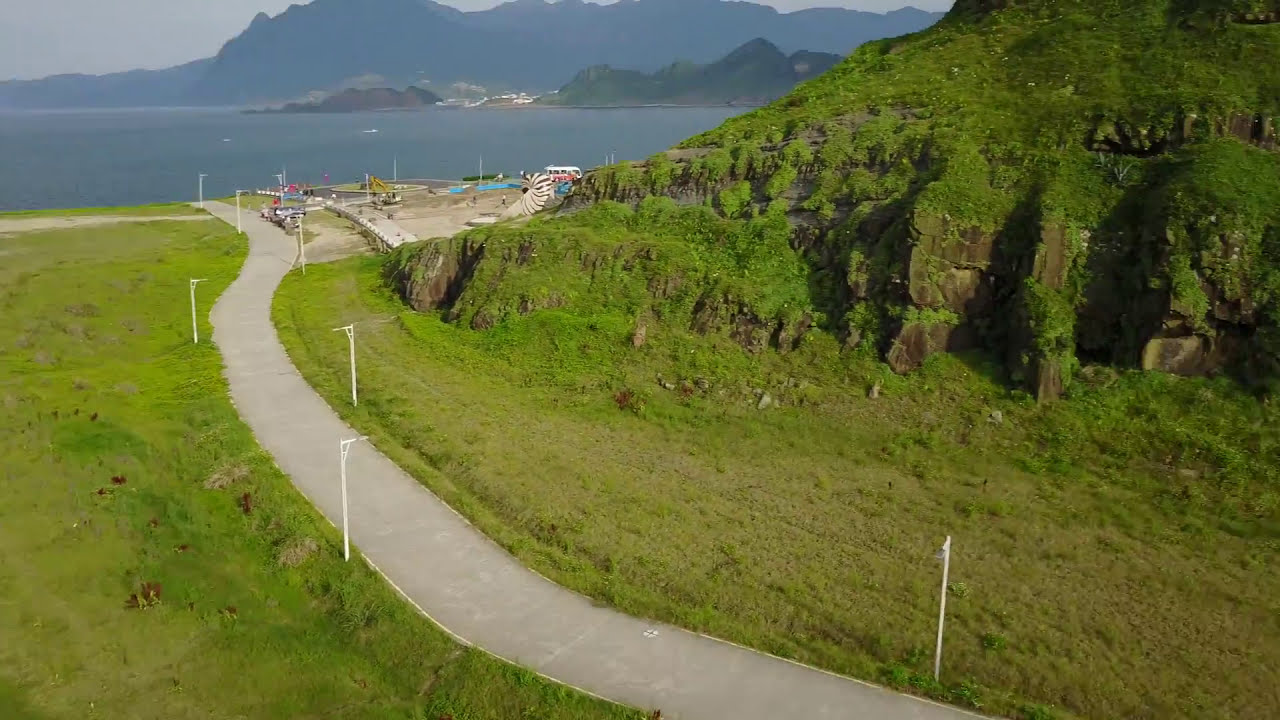This photograph captures an aerial view of a picturesque mountainous region, dominated by a winding, grey asphalt path that cuts through the lush green landscape. The road originates from the base of a verdant mountain on the right, featuring moss, trees, and rocks, and is lined on both sides with white lampposts. As the road curves and extends towards the upper left side of the image, it leads to a sprawling blue body of water, possibly a sea or an ocean. There are a few boats dotting the tranquil water, and beyond it, majestic, dark mountains rise in the distant background. To the left of the road, the terrain transitions from green lawns to a dirt-covered commercial area where a few cars are parked. The serene outdoor scene combines natural beauty with a touch of human presence, illustrating a harmonious blend of land, water, and sky.